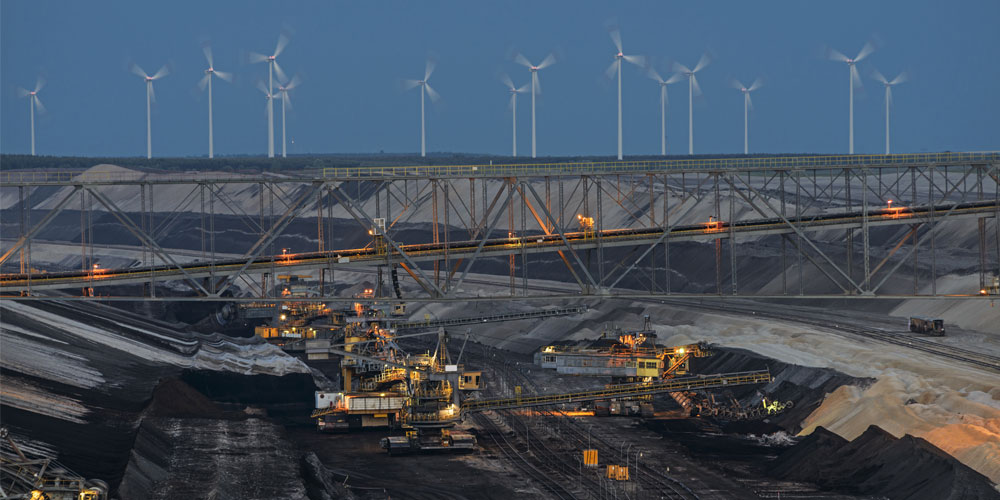The image captures a striking juxtaposition of industrial and renewable energy elements within a dynamic landscape. At the forefront lies a bustling coal mine, its blackish-gray ground marked by mounds of black dirt and several large, yellow vehicles with tank-like wheels, typical of heavy construction and mining equipment. A silver, metal bridge with a V-shaped frame spans the scene, showcasing a grid-style design. Above the coal mine, the sky is a vibrant blue, contrasting the industrious scene below. In the far background, a series of white wind turbines—between 12 and 15—adorn the grassland, their blades in motion, hinting at potential wind energy. The wind turbines are slightly blurred from their movement, indicating their active state. Lights are on both some machinery and a distant building, suggesting that this might be during dusk or night, adding an ambient glow to the busy mining environment.